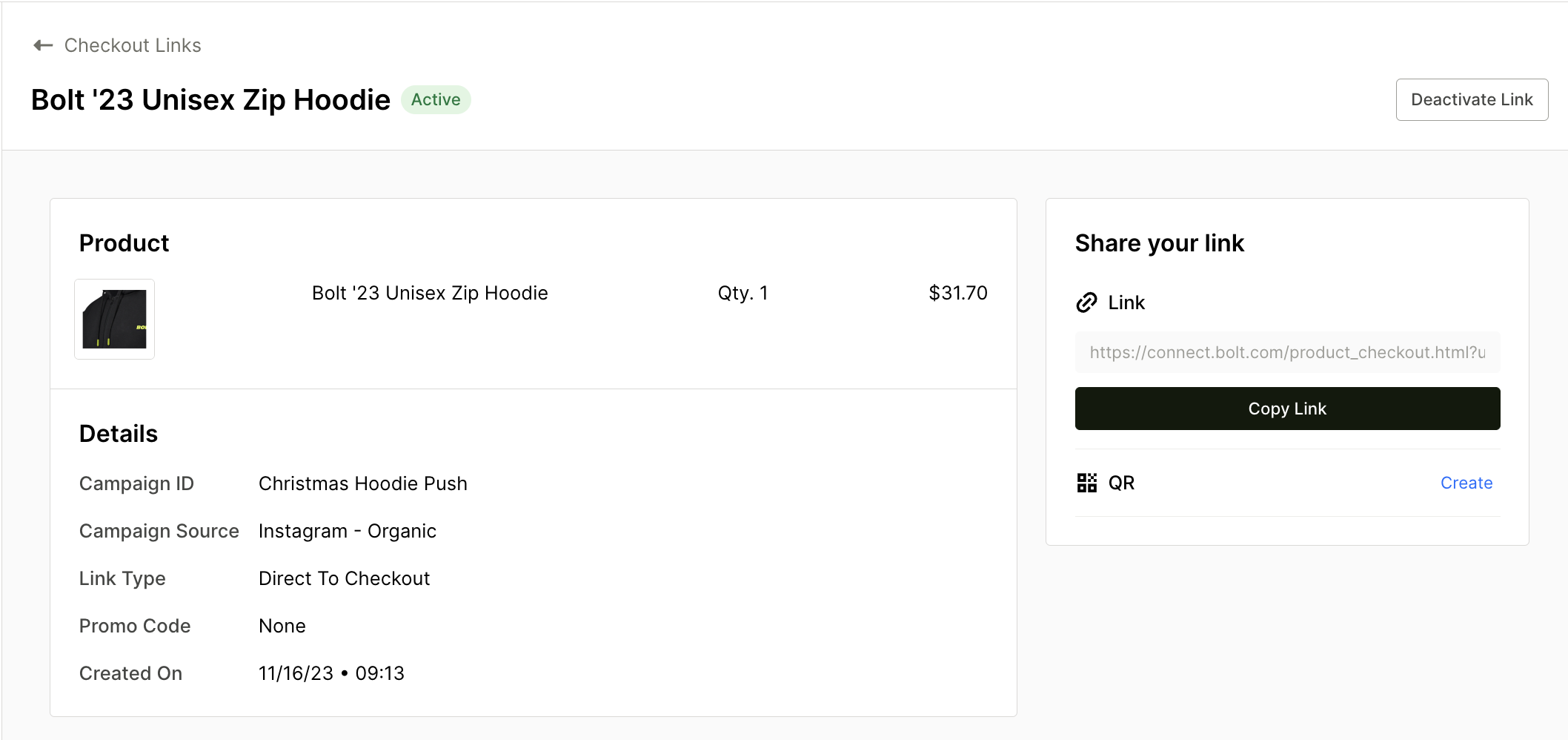The horizontal rectangular image presents a detailed overview of a product listing for an online store. At the top of the image, within a white horizontal box, a black text area prompts users to "Check out links" accompanied by a left-pointing arrow. Below, in bold black font, the text reads "Bold '23 Unisex Zip Hoodie" followed by a light green horizontal oval containing the word "Active" in darker green.

On the far right, there's a horizontal rectangle labeled "Deactivate Link" in black text.

Within the main white rectangular area on the left side, the word "Product" appears in black bold font. Below it, there's an image of the product, which is a black-colored hoodie. To its right, the product name "Bold '23 Unisex Zip Hoodie" is repeated. 

Further to the right, details include:
- **QTY:** 1
- **Price:** $31.70

Below this section, more information is listed:
- **Details** (in bold black font)
  - **Campaign ID:** Christmas Hoodie Push
  - **Campaign Source:** Instagram-organic
  - **Link Type:** Direct to Checkout
  - **Promo Code:** None
  - **Created On:** 11/16/23 09:13

The right side of the page features a section titled "Share your link" in bold black text, accompanied by a paperclip icon and the word "Link." Below, a black horizontal rectangle with white text prompts users to "Copy Link."